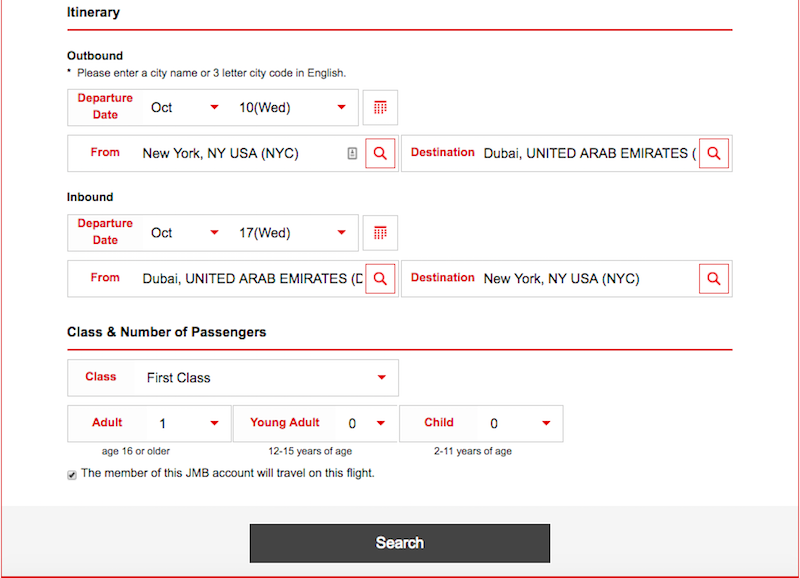**Screenshot of Flight Itinerary on Computer Screen**

The image displays a detailed flight itinerary screenshot from a computer. In the top left corner, the word "Itinerary" is prominently displayed in black. Encasing the main information is a distinct red-bordered rectangle. 

### Outbound Flight Details:

- **Heading**: Outbound
- **Prompt**: "Please enter a city name or three-letter city code in English."
- **Departure Date**: October 10, Wednesday
- **Origin**: New York, New York, USA (NYC)
- **Destination**: Dubai, United Arab Emirates
- **Question Mark Icon**: Located next to the destination in a small box.

### Inbound Flight Details:

- **Heading**: Inbound
- **Departure Date**: October 17, Wednesday
- **Origin**: Dubai, United Arab Emirates
- **Destination**: New York, New York, USA (NYC)

### Passenger and Class Information:

- **Class**: First Class
- **Number of Passengers**:
  - Adult: 1
  - Young Adult: 0
  - Child: 0
- **Drop-Down Arrows**: Each category has a clickable arrow for adjustments.
- **Definitions**:
  - Adult: 18 or older
  - Young Adult: 12 to 15
  - Child: 2 to 11

### Additional Information:

- **Membership Confirmation**: "The member of this JMB account will travel on this flight."

At the very bottom center, there is a long black search bar with the word "Search" displayed in white.